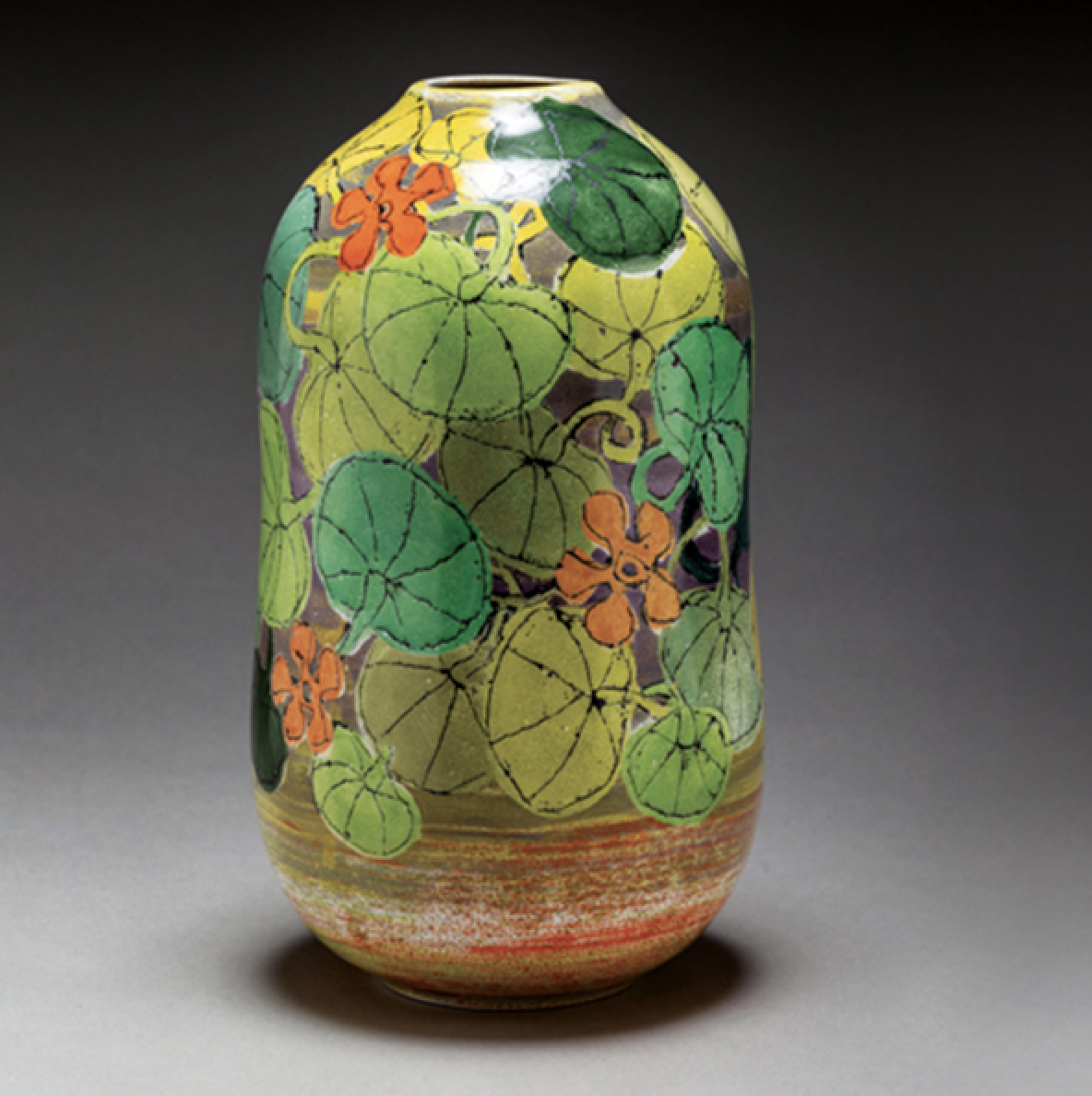The image depicts an intricately designed, tall and slender vase, resembling an urn, with a distinctive Japanese style. Handcrafted and potentially pewter, the vase features a bottom band with faded stripes of yellow, brown, and orange, giving it an aged, weathered appearance. Dominating the main body is a vibrant and varied botanical motif, possibly water lilies or lotuses, captured in overlapping hues of olive green, bluish green, and yellow-green. Scattered among this lush foliage are three vivid orange flowers, each uniquely positioned. The vase tapers gracefully to a smaller, round opening at the top, and its artistic flair suggests it could be an exquisite creation from a pottery studio, perhaps reminiscent of those found in Colorado. The vase rests on a white and gray table, completing the scene.